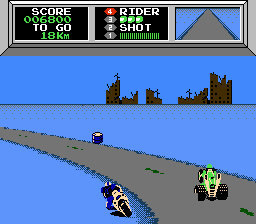The image is a screen grab from the NES video game Mach Rider, featuring a detailed, retro-styled racing scene. In this perfectly square frame, two vehicles race along a curved gray road against a backdrop of a ruined cityscape silhouette. One vehicle is a yellow motorcycle with a rider in black attire and a white helmet with a black stripe, positioned slightly off-road on the left, seemingly bending to the left. The other vehicle is a yellow race car, driven by a character in a green helmet, visible on the road with wide back tires. Blue dominates the ground around the road, with a small blue barrel on the roadside. Above the scene lies an informational rectangle displaying the score, rider info, and attributes. The road features three or four black centerline marks, guiding the racers as they navigate the course.